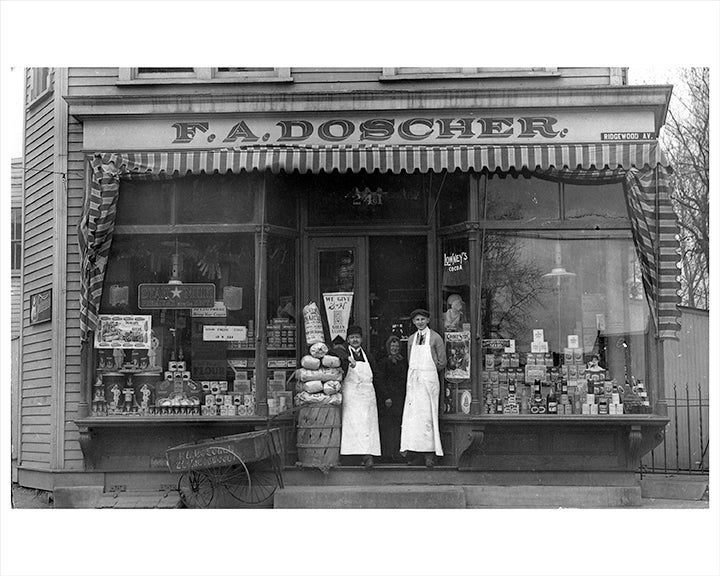This rectangular, black and white photograph, appears to be a photograph of an old photograph, surrounded by a white border. It captures the façade of a historical building, prominently featuring a sign that reads "F.A. Docher. Ridgewood AV" at the top. Beneath this sign, an awning with dark and light stripes is retracted, revealing the entrance of what seems to be a general store. 

At the doorway, two men stand facing the camera, both dressed in long white aprons, hats, and ties, indicating their role as workers or proprietors of the store. The man on the left is noticeably shorter than the man on the right. To the left of the entrance, a large barrel of goods stands, suggesting the store’s trade in various commodities. The storefront includes extensive display windows, showcasing an array of items inside, pointing to the diverse merchandise available within the store. Additionally, a small cart is positioned on the bottom left-hand side of the photograph, adding to the historical ambiance of the scene.